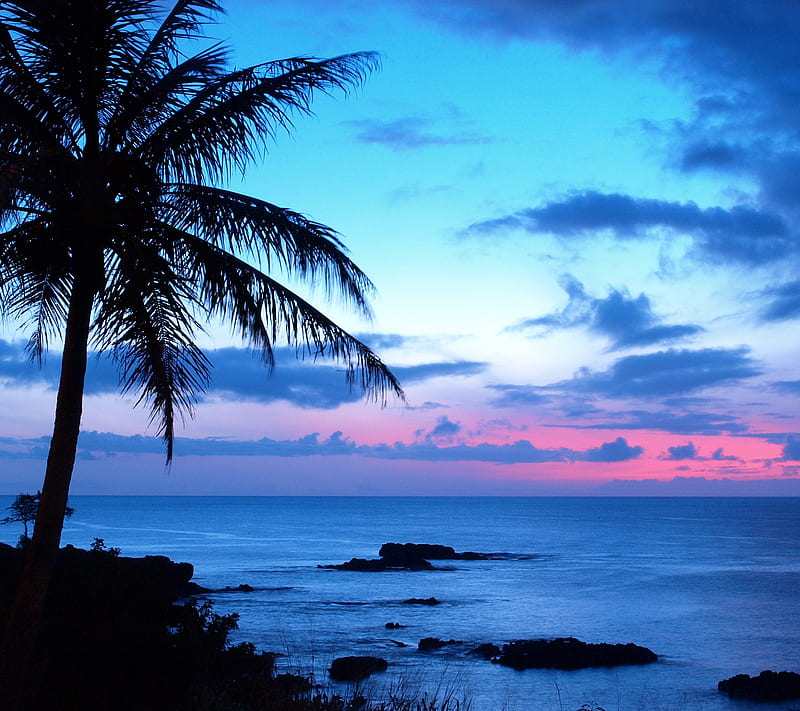This captivating outdoor photograph depicts a serene tropical sunset. Dominating the bottom left corner, a tall palm tree with expansive, arching fronds stands completely silhouetted against the vibrant backdrop, alongside a similarly darkened shoreline and rocky outcrops. The ocean, stretching across the middle ground, reflects the sky's evolving palette, remaining remarkably calm with minimal waves. In the bottom center and right, a few rocky protrusions emerge from the water, adding textural interest.

The sky is a mesmerizing gradient, transitioning from a vivid pink and purple near the horizon on the right to a paler, lighter blue at the top, punctuated by darker blue, puffy clouds. The convergence of these colors suggests that this is indeed a sunset scene, with the sun having just dipped below the horizon, casting the entire landscape in a tranquil, ethereal glow. The horizon, marked by an endless expanse of open ocean, intensifies the sense of peace and natural beauty.